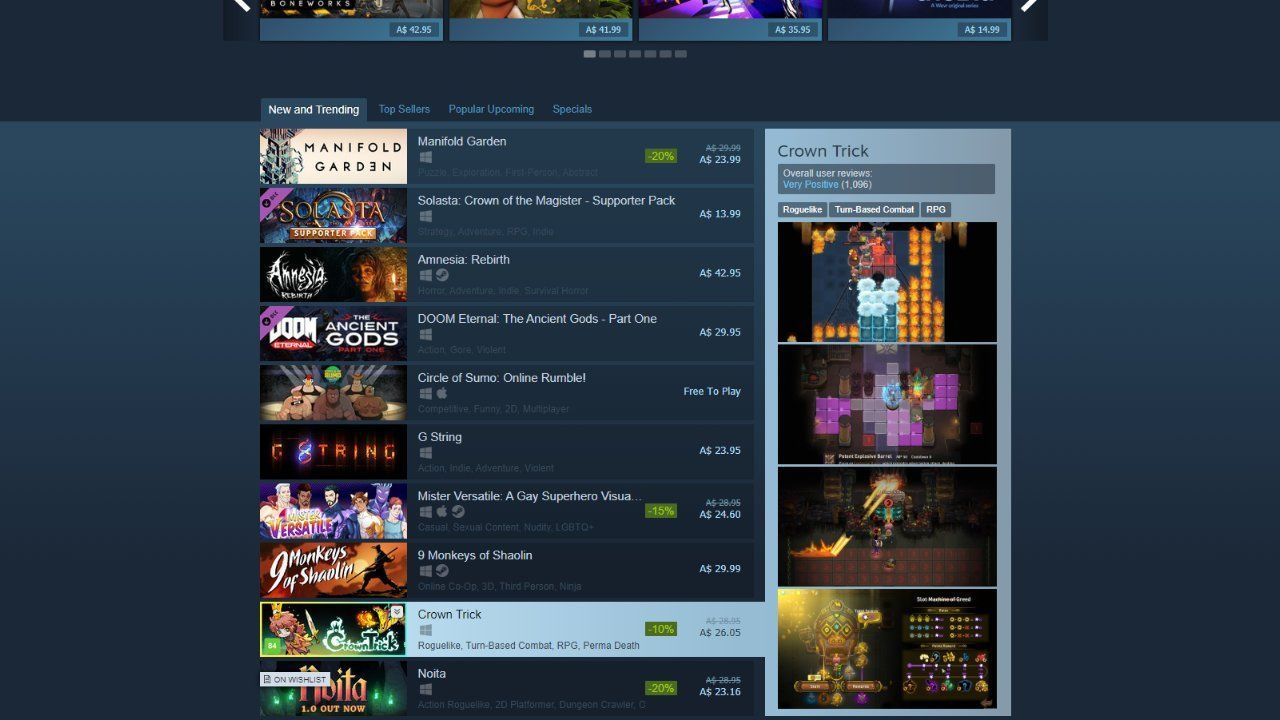This vibrant and detailed image features a variety of game advertisements, each with unique displays and pricing:

- To the left, within a white box, the game "Manifold Garden" is prominently featured.
- Adjacent to it in a small green box is a discount of "20%," making the price "$23.99."
- Below this, "Solasta, Crown of the Magister - Supporter Pack" is listed at "$13.99."
- Continuing downward, "Amnesia" is priced at "$42.05."
- Next, "Doom: The Ancient Gods, Part 1" is highlighted at "$29.95."
- Further down, the game "Circle of Sumo" is mentioned.
- Below that, another game titled "G-String" appears.
- Following in the sequence, "Master Versailla: Nine Monkeys of Shaolin" is indicated.
- In a blue background, the words "Crown Trick" are displayed, accompanied by a small animated cat to the left.
- Finally, at the bottom, the game "Noita" is shown with bright green lines on each side of the title.

On the right side of the image, at the top of the next box, "Crown Trick" is again listed. Below this, there appears to be a complex visual resembling a Tetris game with numerous gold circles arranged within a graph-like structure.